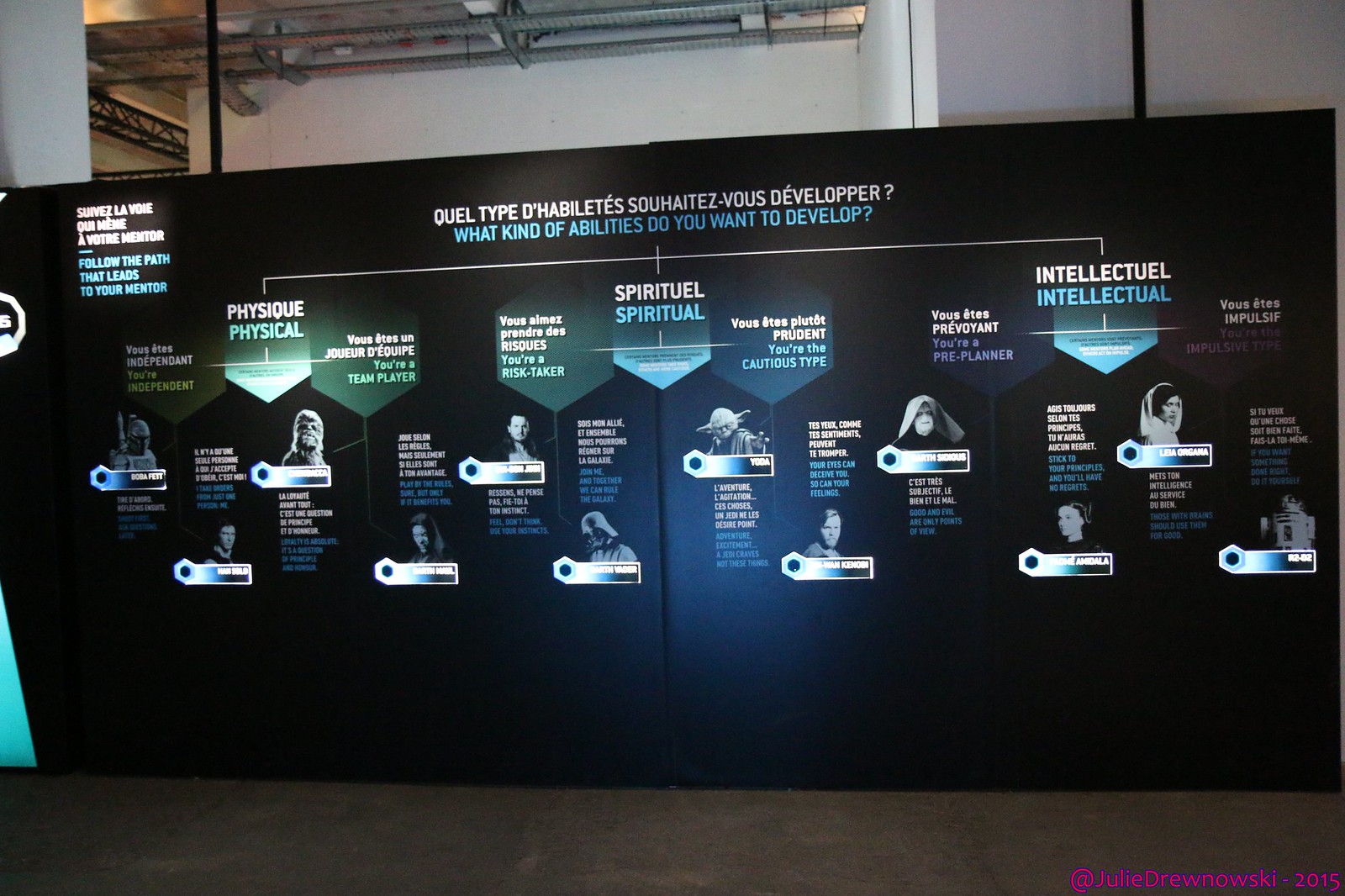The image depicts a large, horizontally-aligned rectangular display wall at an indoor event, possibly a museum. The wall features characters from Star Wars and is split into three sections, each representing different types of abilities: Physical, Spiritual, and Intellectual. At the top, the text "What kind of abilities do you want to develop?" is displayed in both French (white text) and English (blue text). Under each category, various Star Wars characters are positioned, including Chewbacca under Physical, Yoda under Spiritual, and Princess Leia under Intellectual. Additional characters such as the Emperor, Princess Amidala, and R2-D2 are also arranged within their respective sections. The display is set against a backdrop of other similar walls and a white ceiling. The sign contains detailed descriptions and labeling in both languages, with relevant text such as "physique, physical," "spirituel, spiritual," and "intellectuel, intellectual" guiding viewers. At the bottom right corner of the display, the text "@Julie Drunoski, 2015" is visible, and the overall color palette includes shades of black, white, blue, green, purple, gray, and silver. Stone flooring can be seen at the bottom of the image.